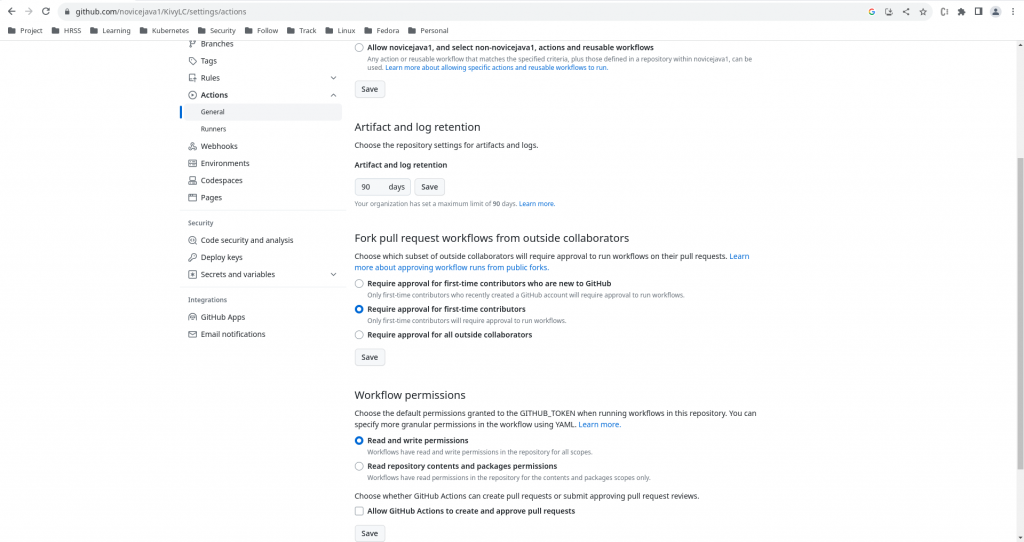The image showcases a webpage with various interface elements against a white background:

1. **Top Navigation Bar**:
   - Contains a left arrow, a right arrow (grayed out), and a refresh icon.
   - An address bar with a lockpad icon and a web address displayed in gray.
   - Icons for Share, Favorite, and Google.

2. **Horizontal Menu**:
   - Lists different categories including Project, HRSS, Learning, Kubernetes, Security, Follow Track, Linux, Fedora, and Personal.

3. **Center Content**:
   - Displays multiple sections including Branches, Tags, Rules, Actions, General, Runners, Webhooks, Environments, Codespaces, Pages.
   - Additional sections like Security (Code Security and Analytics), Deploy Keys, Secrets and Variables.
   - Integration settings with GitHub Apps, Email Notifications, and options to allow novice and non-novice Java actions.

4. **Footer**:
   - Contains a "Save" button.
   - Information on artifact retention for 90 days, work pool settings, requests for workflows from outside collaborators, and workflow permissions.

Overall, the image appears to be a detailed snapshot of a website's user interface featuring extensive navigation and functional options across various sections.